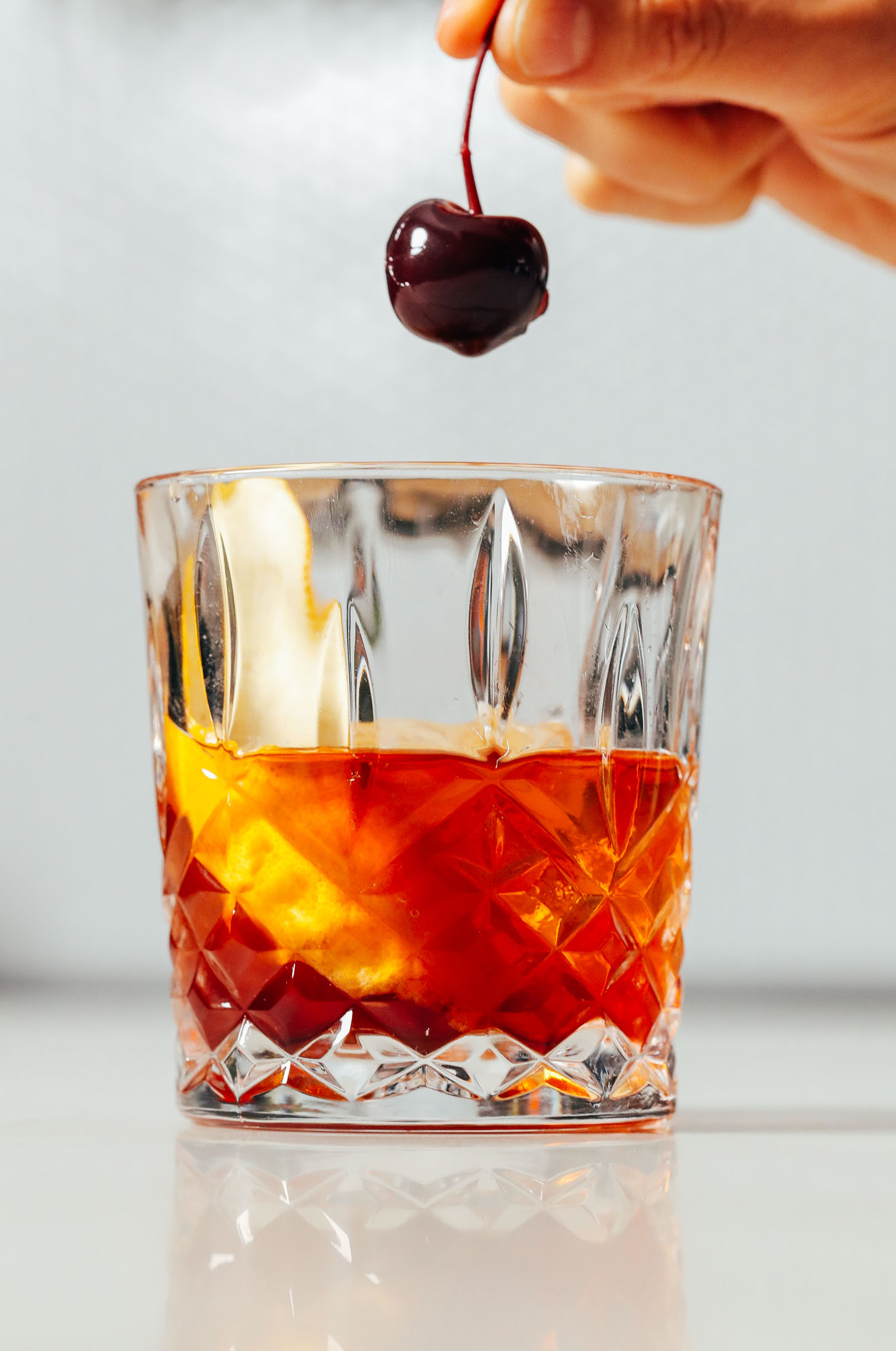This vivid color photograph captures the moment a person is about to drop a bright red cherry into a meticulously crafted Old-Fashioned cocktail. The drink, bathed in a rich orange-brown hue, stands in the center of a reflective, shiny table, which mirrors the glass and its contents. This carefully mixed cocktail, encased in a fancy, cut crystal rocks glass, contains a slice of lemon and a wedge of lime, adding a zesty, citrus twist to the classic drink. The scene is set against a gray background, with a white wall in sight, enhancing the clarity and detail of the image. In the upper right corner, a hand, with only the thumb and index finger visible, delicately holds the stem of the cherry, poised to dip it into the drink. The photograph’s focus is sharp and clear, revealing even the fine scratches on the glass, capturing the elegance and precise moment of cocktail preparation.